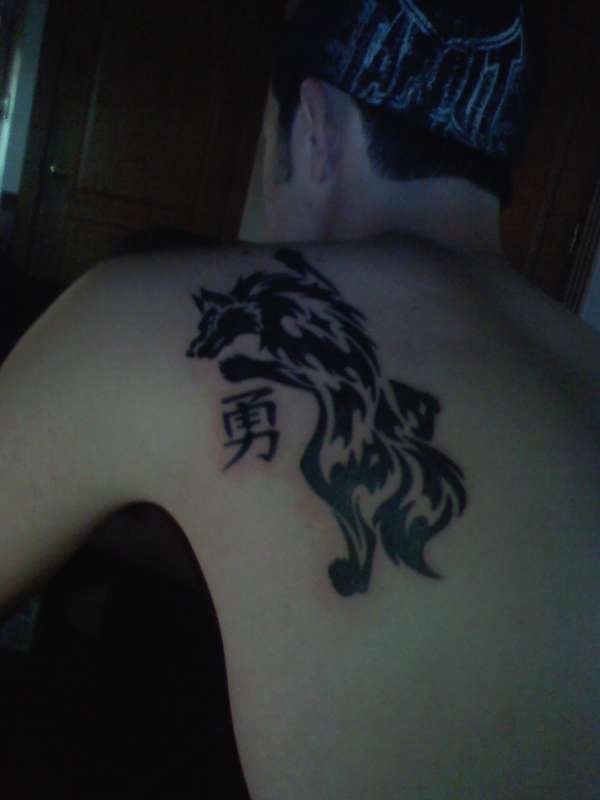This image captures the upper back of a man with short dark hair, featuring notable sideburns in front of his left ear. He appears to be wearing a cap or a handkerchief on his head, though the details are blurred due to the dark and grainy nature of the photo. The man’s shirtless torso showcases a large, intricate tattoo of a wolf on his back, centered prominently. The wolf is depicted standing on its hind legs with its front legs outstretched, giving the impression of it climbing or spreading across his back. The wolf’s head, with ears pointed upwards, is positioned near the man’s left shoulder, gazing to the left. The tattoo is stylistically designed with areas of skin showing through, mimicking the texture of fur. Below the wolf’s left front paw, there's a Chinese or Japanese character, set against a slightly irritated, pinkish background, suggesting the tattoo might be relatively new. The backdrop of the image is dim, but a dark brown door is faintly visible, indicating that the photo was taken in a low-light setting, possibly at night.